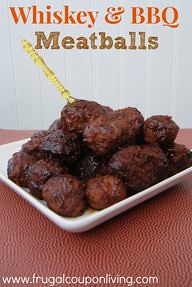This vertical rectangle image, resembling a flyer, magazine cover, or poster, features a realistic photograph of a culinary dish. The background displays vertical wooden planks painted light blue, and the lower section presents an orange or reddish surface, likely a table or tablecloth. In the center, a shallow, white, squarish plate holds a pyramid of approximately 20 to 30 dark brown, juicy meatballs covered in barbecue sauce. A golden fork is elegantly sticking out from the top meatball. At the top of the image, bold red or orange text reads "Whiskey and BBQ," followed by "Meatballs" in brown text. The bottom left corner features the website "www.frugalcouponliving.com" in white text, emphasized across the orange surface.